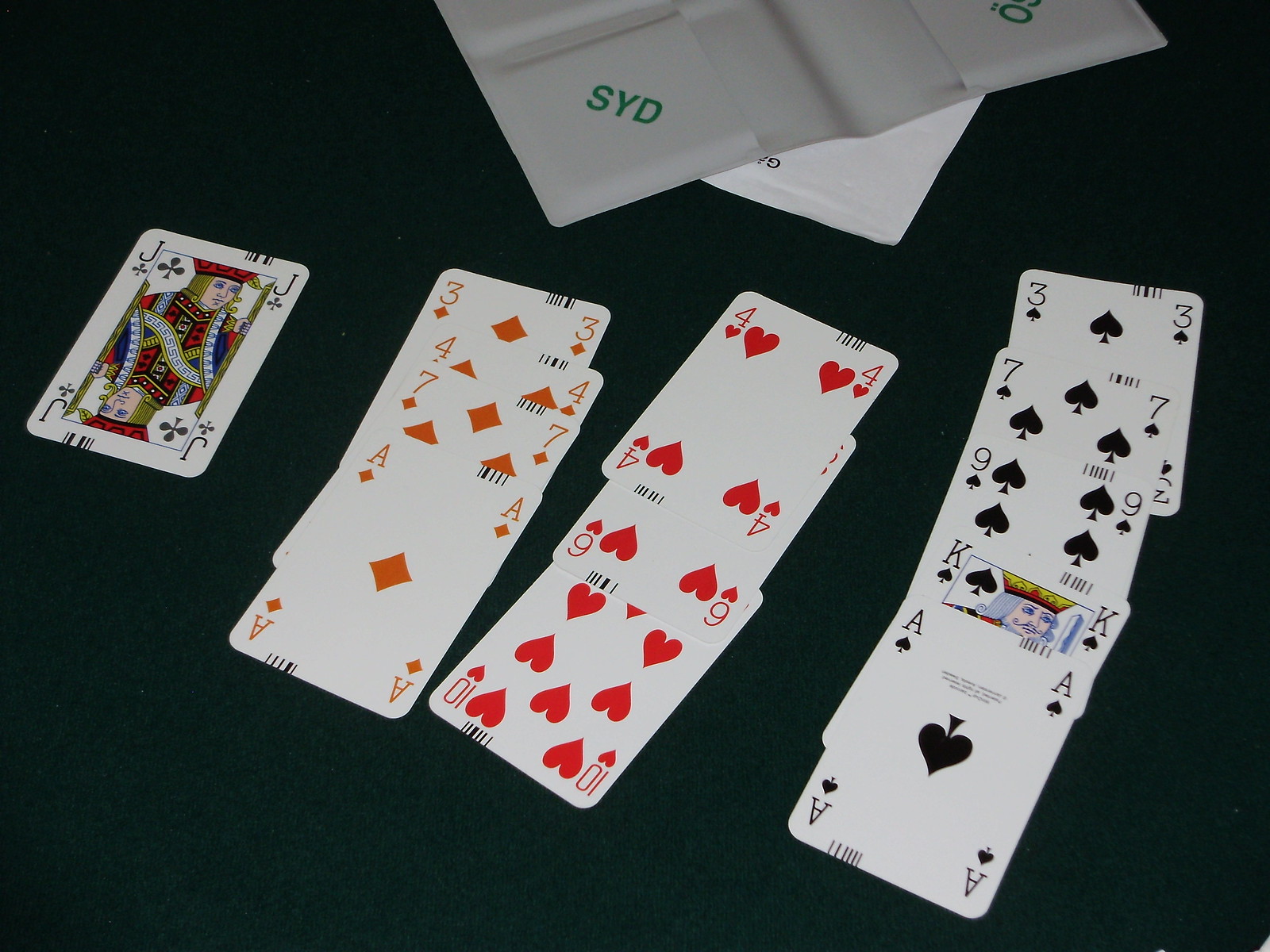The photograph showcases a meticulously arranged collection of playing cards against a jet-black background, evoking an ambiance akin to a solitaire game in progress. To the left, the sequence begins with a solitary black Jack, exuding an air of singular importance. Adjacent to the Jack is a spread of diamond-suited cards: a Three of Diamonds on top, followed by a Four of Diamonds, a Seven of Diamonds, and at the bottom, an Ace of Diamonds. 

Progressing rightwards, the next organized stack is topped by a Four of Hearts, under which lies a Six of Hearts and a Ten of Hearts, revealing a red suit theme. To the far right, a column of spades asserts its dominance with a Three of Spades at the top. This pile descends through a Seven of Spades, a Nine of Spades, a King of Spades, and finally culminates in an Ace of Spades.

Positioned at the top of the composition are two overlapping white objects. The topmost appears to be a piece of plastic packaging, emblazoned with the letters "S.Y.D.", while the one beneath it seems to be another flat, white paper-like item, adding an enigmatic element to the scene. The contrast of the cards against the dark backdrop and the scattered white objects above them creates a visually captivating tableau.